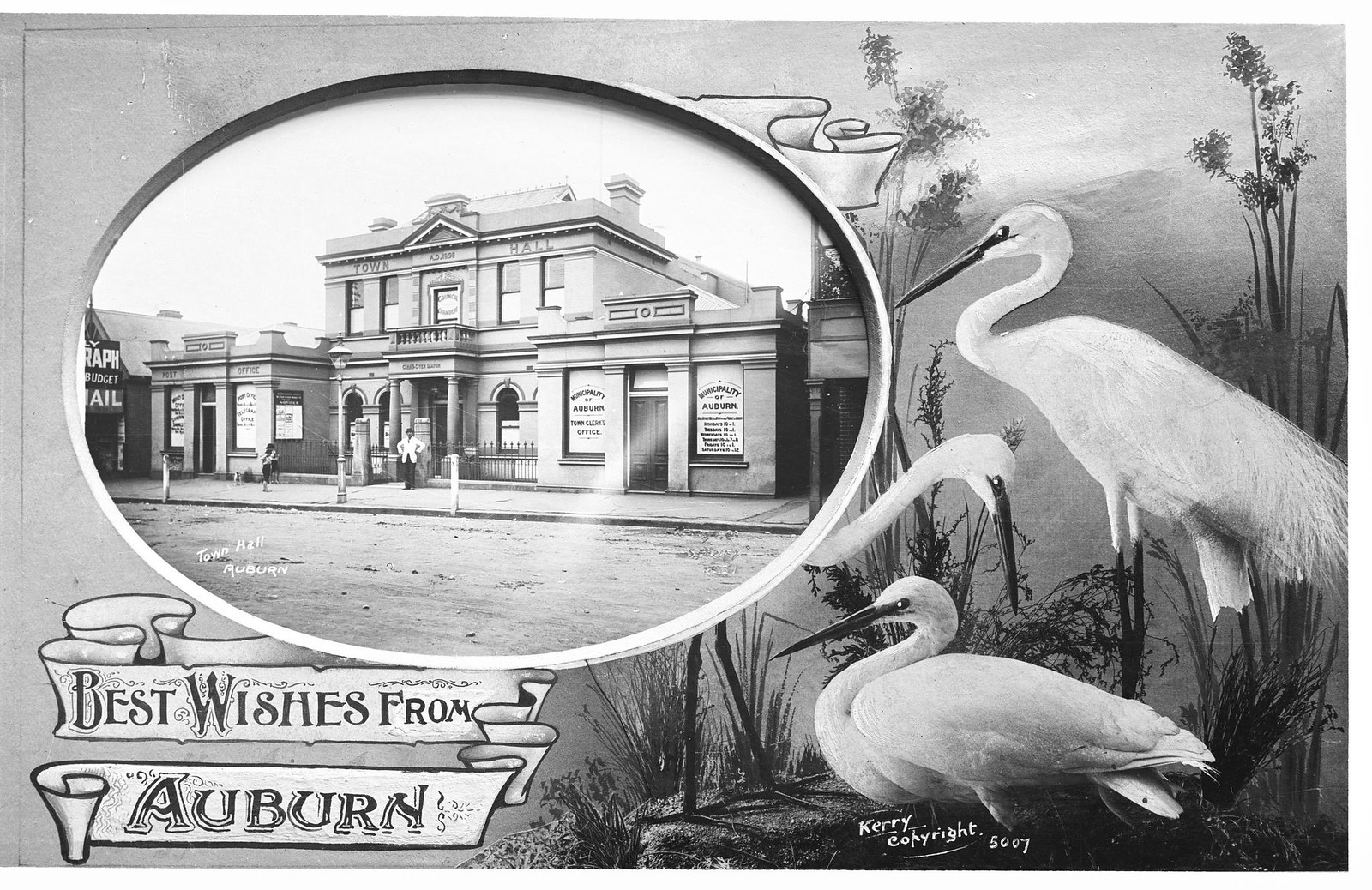The image is a rectangular postcard, wider than it is tall, presented in black and white. In the upper left quadrant, there's an oval-shaped photograph depicting an old black-and-white scene of the Town Hall in Auburn. The Town Hall building, marked with "A.D. 1898" at the center top, is two stories high, flanked on the left by a Post Office and on the right by an office marked "Municipality of Auburn Town Clerk's Office." In front of the Town Hall stands a man wearing a white dress jacket, a hat, and black pants, with his hands on his hips. Below this photograph, in the lower left segment of the postcard, is a banner reading "Best Wishes from Auburn."

On the right side of the postcard are images of three storks (described as swans in some accounts), with varying positions: one is seated on the ground, another shows just its neck, and the third is standing. Near these bird images, in the bottom right corner, is the signature "Carrie, Copyright 5007."

Overall, the postcard combines historical architecture with natural scenery, framed by additional decorative elements such as flowers, grass, and water features, creating an intricate and nostalgic visual.